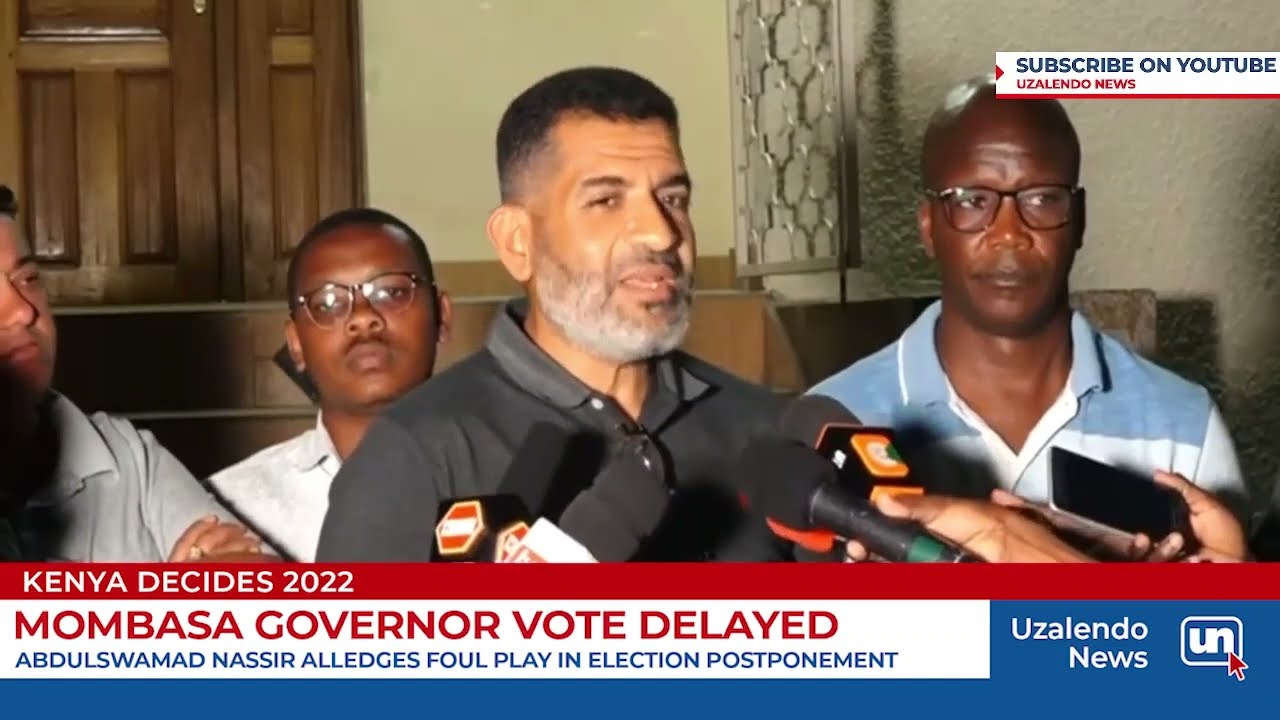The image is a detailed screen grab from a color news broadcast titled "Kenya Decides 2022." At the center, a man with dark brown hair styled in a crew cut and wearing a black polo shirt speaks into several microphones positioned near his mouth. Surrounding him are three gentlemen, two of whom are African-American men with glasses. One wears a white collared shirt with folded arms, and the other sports a white and blue shirt. The third man, visible only partially, is also wearing glasses and an expressionless face. Behind them is a backdrop of a chapel or building adorned with stained glass windows and dark wood paneling, setting a somber tone to the scene.

The chyron at the bottom of the screen reads in red, "Kenya Decides 2022," and in white beneath it, "Mombasa governor vote delayed. Abdul Swamad Nasir alleges foul play in election postponement." The lower right corner features the "Yuzalindo News" logo accompanied by a UN logo in a bold sans-serif lowercase font. Additionally, a prompt in the upper right corner encourages viewers to "subscribe on YouTube." This carefully framed image captures a tense moment, emphasizing the serious atmosphere surrounding the election issues in Mombasa.